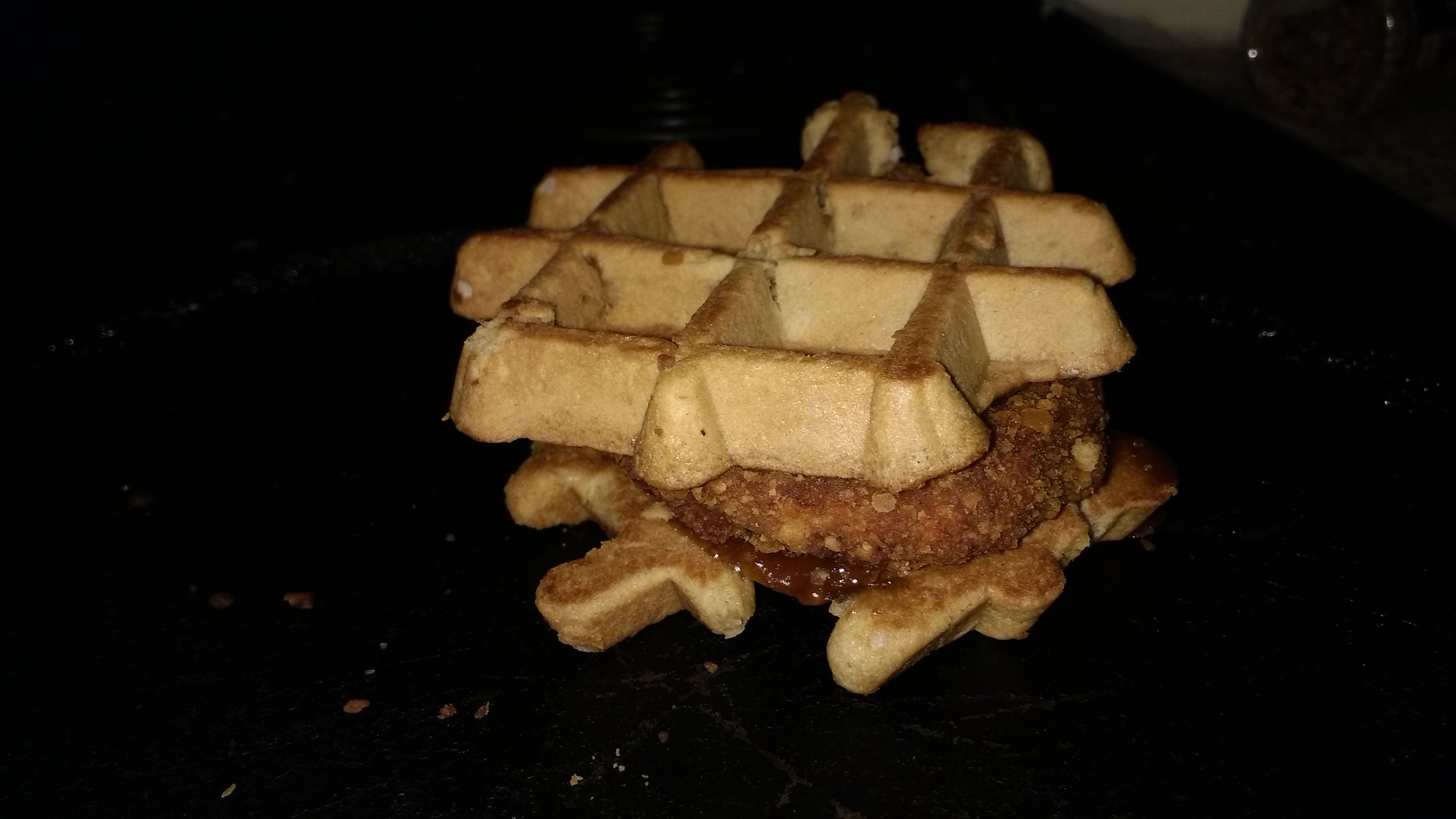The photo showcases a waffle sandwich on a dark surface, possibly a black pan or table. The sandwich consists of two thick, light tan waffles with large square indents and dark brown, toasted edges. Nestled between the waffles is a dark brown, crumbly textured strudel with a thick, gooey tan or orange filling oozing out. Some descriptions suggest the possibility of it being a piece of chicken or sausage with a syrup-like sauce. The background reveals a gray granite countertop with a plastic bottle on the right, adding to the impression of a restaurant setting. The photograph, taken under dim lighting, emphasizes the messy yet appetizing look of the dish.